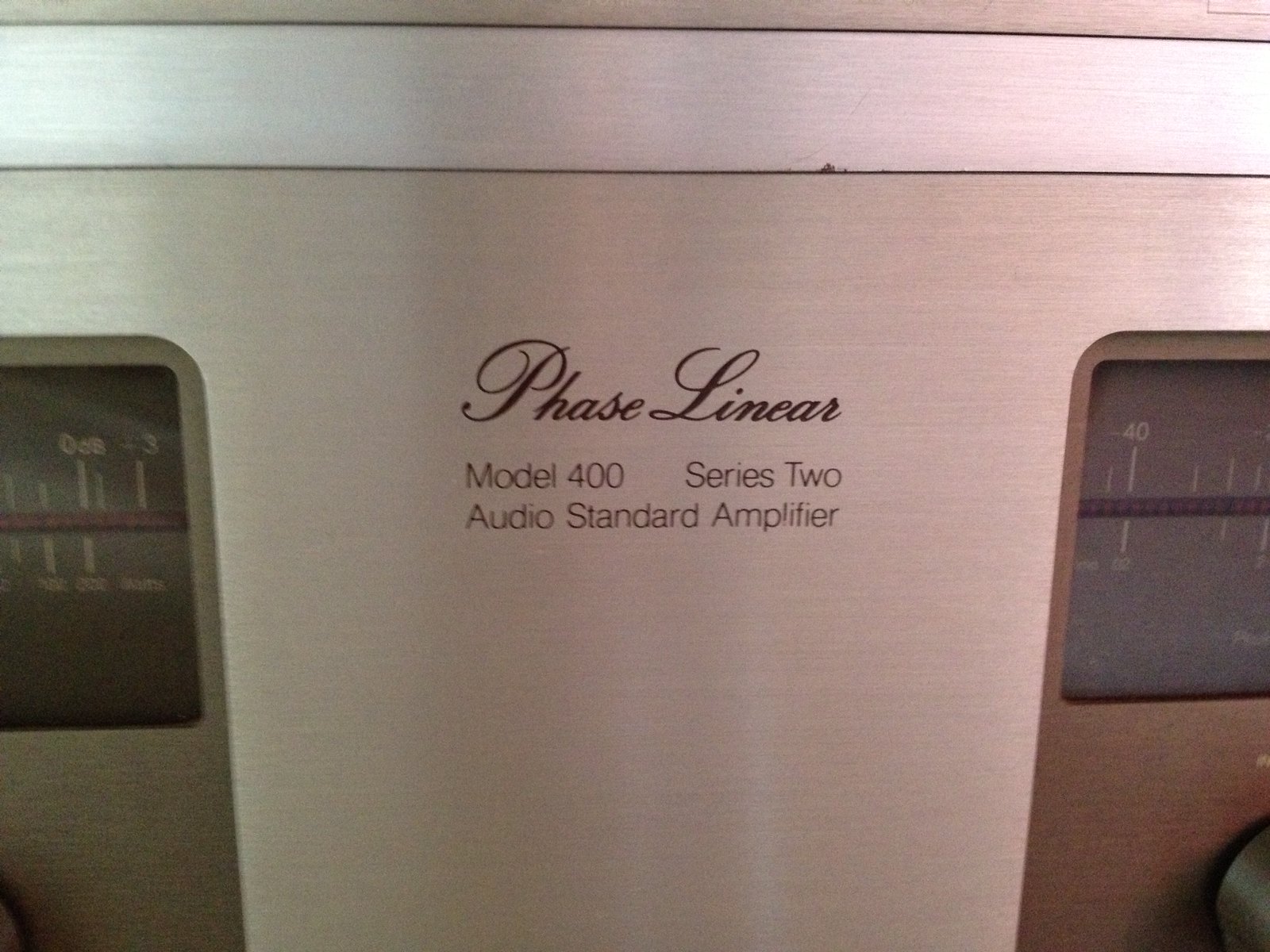This is a close-up photo of a polished, high-end, stainless steel Phase Linear Model 400 Series 2 Audio Standard Amplifier. The amplifier prominently features a middle metal section with cursive black print stating "Phase Linear," and non-cursive black print below it specifying "Model 400 Series 2" and "Audio Standard Amplifier." On either side of this central section are two analog screen panels; the left screen displays "-3," although part of it is cropped out, while the right screen shows the number "40" with a circular knob below it. There are additional dials and numbers on these screens, possibly indicating input levels or frequency adjustments, typical of audio equipment. A silver stripe runs along the top of the amplifier, and the material's high-quality construction adds to the premium appearance of the device. The image appears slightly curved due to lens distortion.